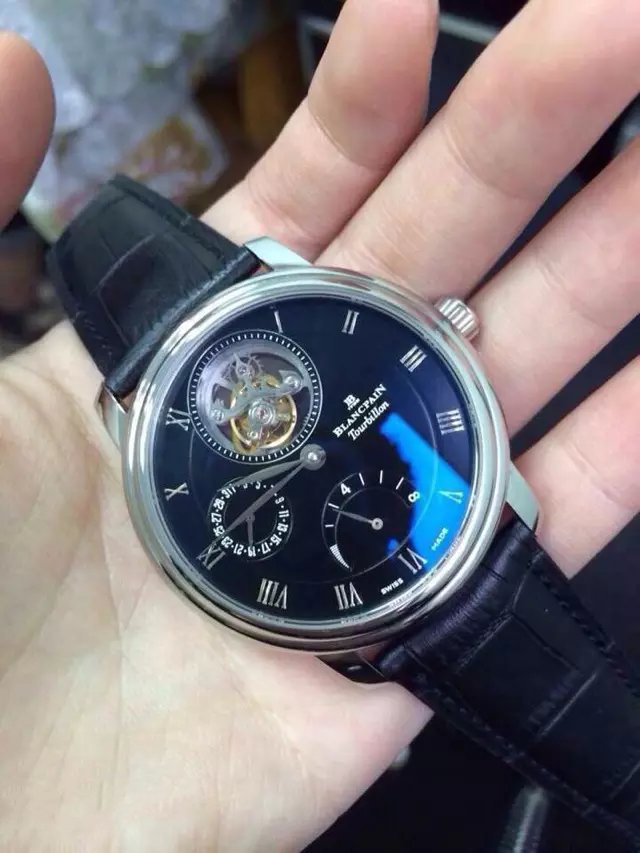The image depicts a close-up photograph of a luxurious Blancpain Tourbillon watch resting in the pale, left hand of an individual with white skin. The watch features a sleek, silver housing and a dark blue face adorned with silver Roman numerals from I to XII. Notably, the face also showcases an intricate mechanism exposed at the center top, revealing part of the inner workings of this high-end timepiece. The hands of the watch include two additional sub-dials or indicators. A reflection on the watch’s glass indicates its high-quality craftsmanship. The watch is secured with a black leather band, likely made from alligator or crocodile leather. The background is lightly visible, showing mostly medium browns and greyish hues.